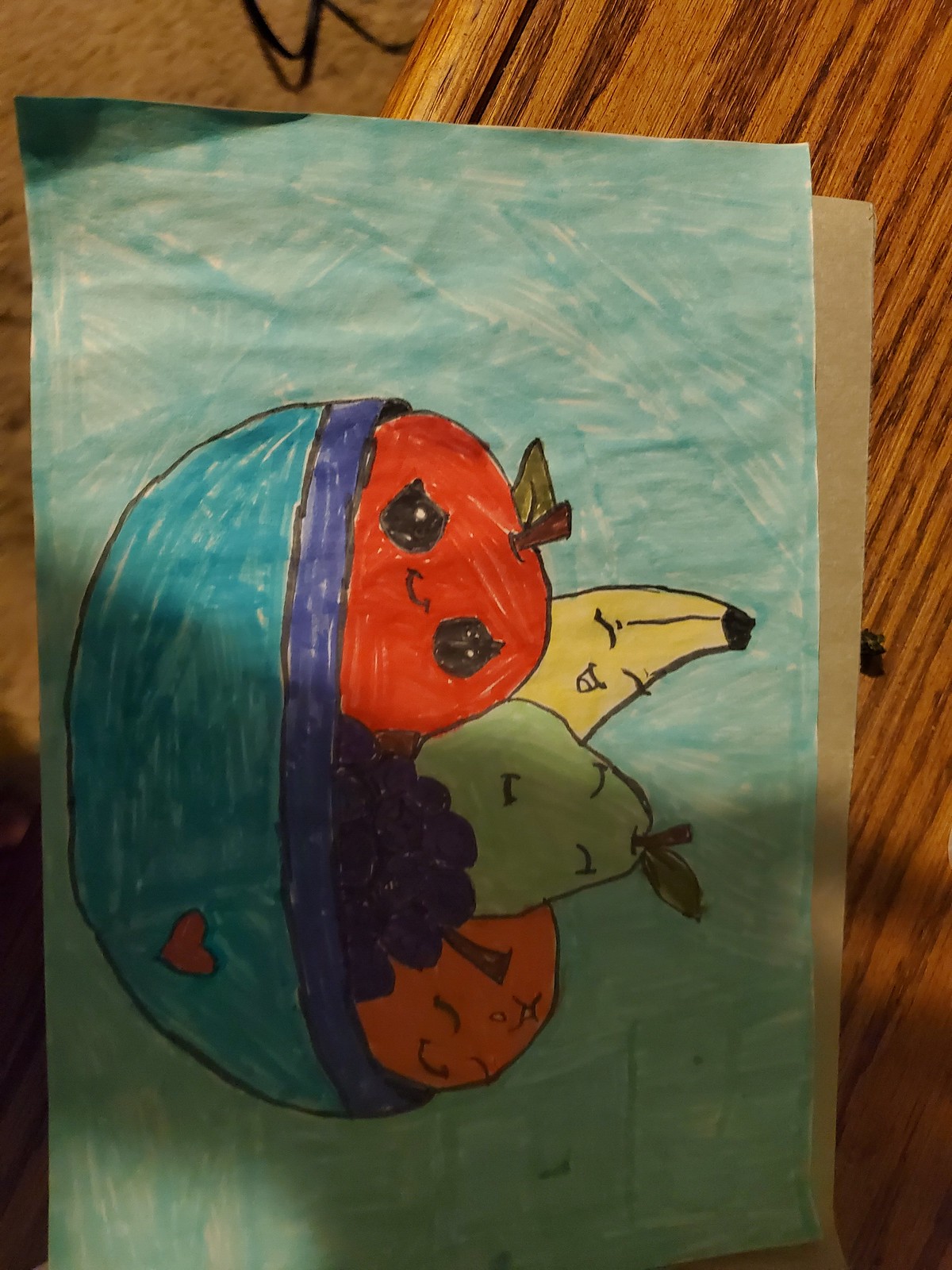This is a photograph of a child's drawing, rendered in marker. The drawing showcases a whimsical bowl of fruit, each piece adorned with charming cartoon faces. The fruit ensemble consists of a red apple, a yellow banana, a green pear, a cluster of purple grapes, and an orange. The expressions of the fruit are delightfully varied, with some having open eyes and others with eyes closed, all exuding a sense of happiness and contentment. The blue bowl holding the fruit features a darker blue band along the top edge, and a small heart is drawn on the bowl, adding a touch of warmth. The background of the image is a turquoise color, complementing the playful theme. The drawing is on a medium-brown wooden surface, likely a table or desk, which adds a homely and rustic feel to the presentation.